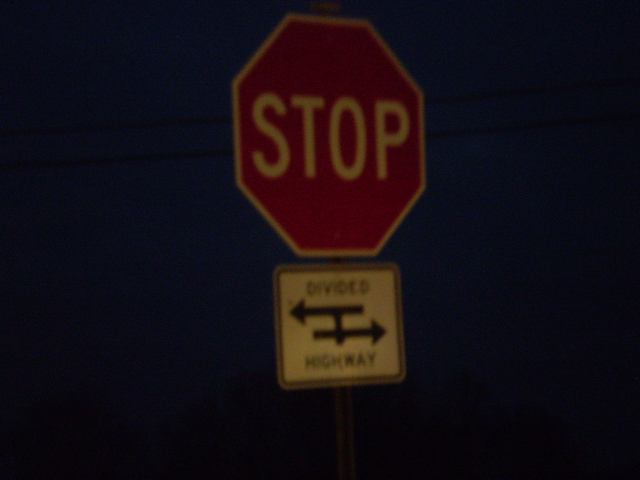The image depicts a standard red octagonal stop sign with another white rectangular sign attached below it, reading "DIVIDED HIGHWAY." The white sign features an outline of two arrows pointing in opposite directions, separated by a lane in the middle. The photograph is evidently taken during the night, under very low light conditions. The background is shrouded in darkness with minimal visibility, showing some indistinct, blurry elements like power lines and possibly trees. The overall scene is quite dark, with a slight yellowish tint and poor focus, suggesting it was captured while driving past the signs.